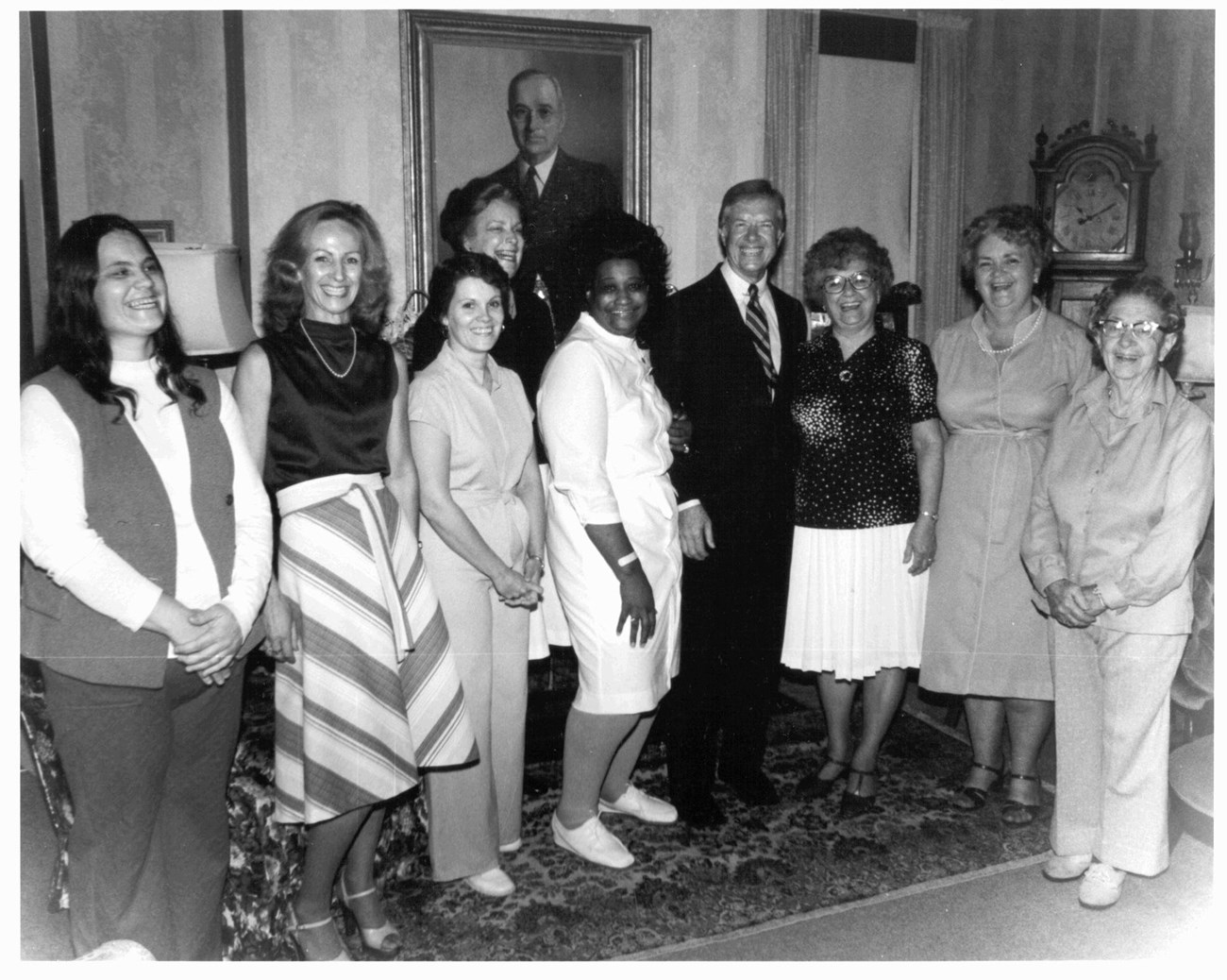This black-and-white photograph, likely from the 1960s or 70s, appears to be taken in an official setting, possibly a museum or the White House. The central figure is President Jimmy Carter, who is dressed in a suit and surrounded by a group of nine women, all smiling genuinely. Among the women, there are predominantly older white women, two wearing glasses, with a mix of dresses and a pantsuit. There is also one black woman in a white dress standing close to President Carter. The background features a framed painting, probably of President Franklin D. Roosevelt or Harry Truman, and an elegant grandfather clock. The group is standing on a Turkish rug, suggesting a formal and significant occasion, possibly a celebration of impactful legislation or an important milestone benefiting women. The overall scene is one of happiness and genuine camaraderie, with everyone dressed formally and exuding authentic joy.